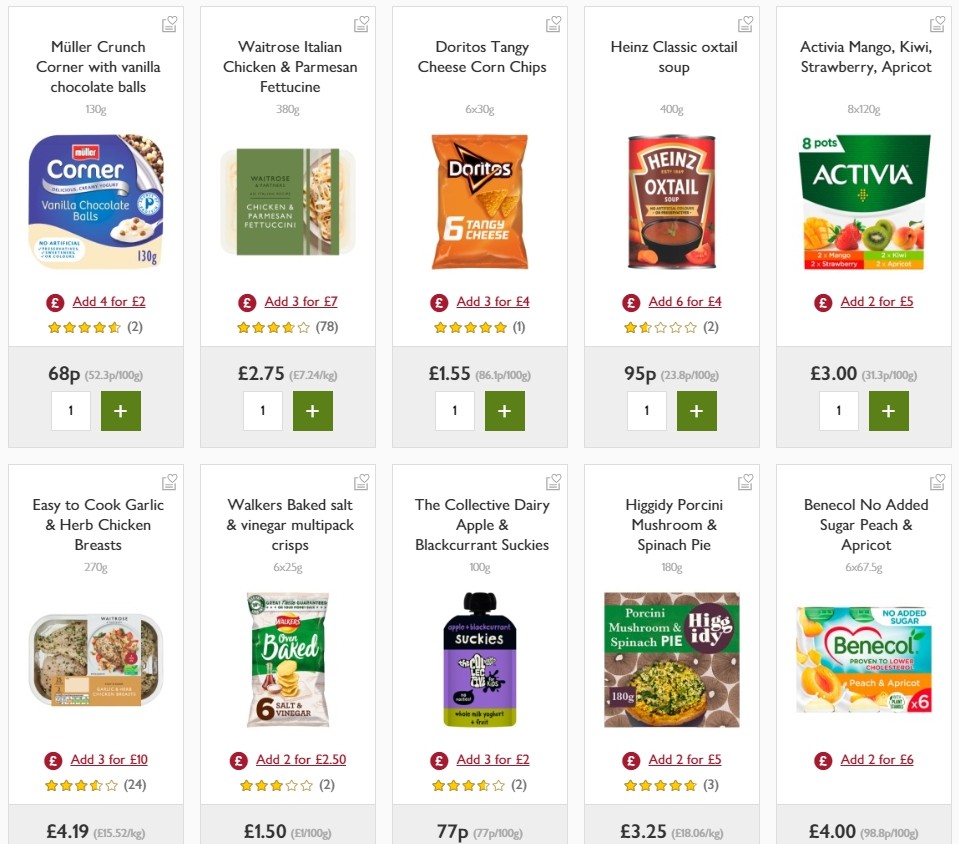This screenshot captures the interface of a grocery store shopping app, possibly from a British retailer, as indicated by the prices listed in British pounds. The display showcases 10 different grocery items, each accompanied by a thumbnail image and a descriptive title above it. Beneath each item title, there is a rating system represented by stars, followed by the item's price. At the bottom of each grocery item entry, there is a button to add the product to the shopping cart. The layout effectively integrates essential shopping details, providing users with a clear and concise summary of each product's image, name, rating, price, and purchase option.